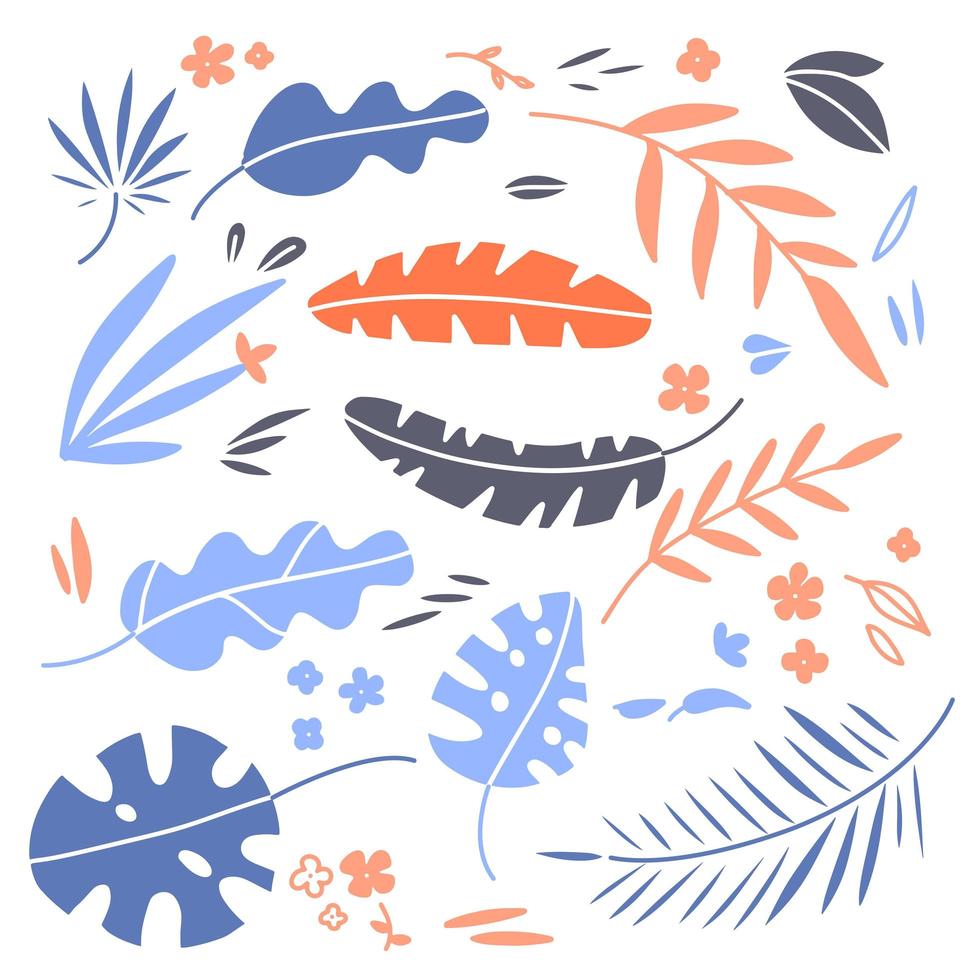The image is a minimalistic and stylized design featuring a diverse array of floating leaves and flowers against a white background. The artwork includes various types of leaves, such as fern-like wispy leaves, monstera leaves with holes, feather-like leaves, and long thin leaves. The colors of the leaves span a range that includes light blue, dark blue, periwinkle blue, light coral orange, dark coral orange, dark gray, and hints of rose gold. Some leaves are solid-colored, while others have intricate line patterns or appear to have clipped or eaten sections. Interspersed among the leaves are small flowers, some with stems and others without, ranging in color from rose gold to blue. One flower, reminiscent of a blue sand dollar, stands out among the design elements. The overall composition is reminiscent of computer clipart and provides a sense of autumnal variety without any textual context or explanation.